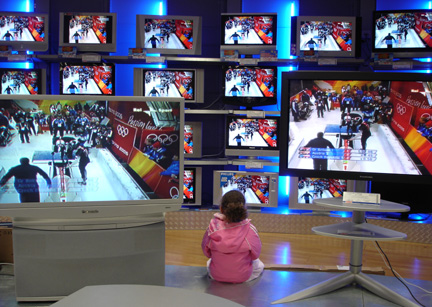In the image, we see a young girl with brown hair tied in a mid-level ponytail, sitting on a light brown wooden floor in the TV section of an electronics store. She is wearing a pink jacket and white bottom clothing, though it is unclear whether it is a dress, skirt, or pants. The focus of her attention is a large display wall filled with around 20 televisions of varying sizes—all of which are tuned to the same Olympic curling event, as evidenced by the Olympic logo visible on the screens. In front of the TV wall, there is a small bench, on which the girl is seated. The scene captures a moment of captivated viewing as she watches the synchronized broadcast in the store.